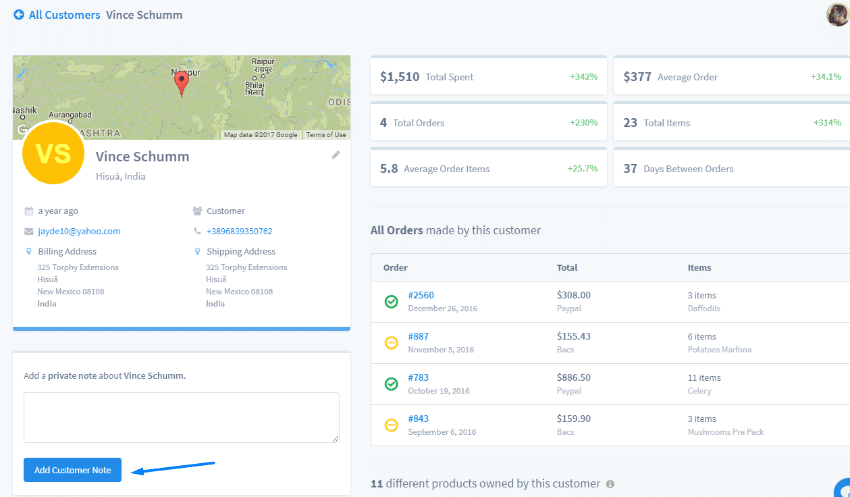This image is a detailed screenshot of a customer dashboard showcasing information about Vince Shum, a user from Hisuwa, India. On the left side of the screenshot, Vince's user profile is displayed, highlighting that he created his profile a year ago. The profile includes his email, phone number, billing address, and shipping address, with his status clearly marked as a 'customer.' There is also an option to add a private note about Vince, with a prominent arrow pointing towards a button labeled "Add Customer Note," suggesting that the image may be part of a tutorial on how to add a customer note.

The central part of the dashboard provides a comprehensive summary of Vince's purchasing behavior, including the total dollar amount spent, the total number of orders, the average cost per order, the number of total items ordered, and the number of days between orders. Except for the last metric, each of these data points also includes the rate of change in percentage.

Underneath these summary statistics is a list of Vince's recent orders, detailing the order number, date of purchase, total amount spent, and the number of items per order. At the very bottom of the dashboard, it is noted that Vince owns 11 different products. The screenshot encapsulates an in-depth view of the customer's order history and profile details, likely serving as a useful tool for customer management and analysis.